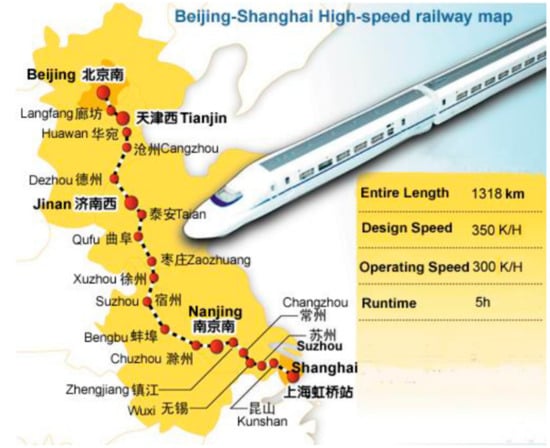This is an infographic-style illustration of the Beijing-Shanghai high-speed railway map, designed to provide detailed information to travelers. The map, drawn in a cartoon-like manner, features a high-speed rail car—white with a gray top and a blue stripe alongside multiple windows—proceeding diagonally from the top right to the bottom left corner. The top section of the map is rendered in white with a light blue corner, while the bottom portion includes a distinct yellow bar highlighting key metrics: the total length of the route is 1,318 kilometers, with a design speed of 350 kilometers per hour, an operating speed of 300 kilometers per hour, and a runtime of approximately five hours. The map depicts the route from Shanghai at the bottom to Beijing at the top, marked with a yellow outline and displaying intermediary stops including Langfang, Huawan, Tianjin, Kangzhou, Dezhou, Jinan, Tian, Tufu, Zhaozhuang, Suzhou, Bengbu, Nanjing, Suzhou, Xinjiang, Wuxi, Kunshan, and Chengzhou.